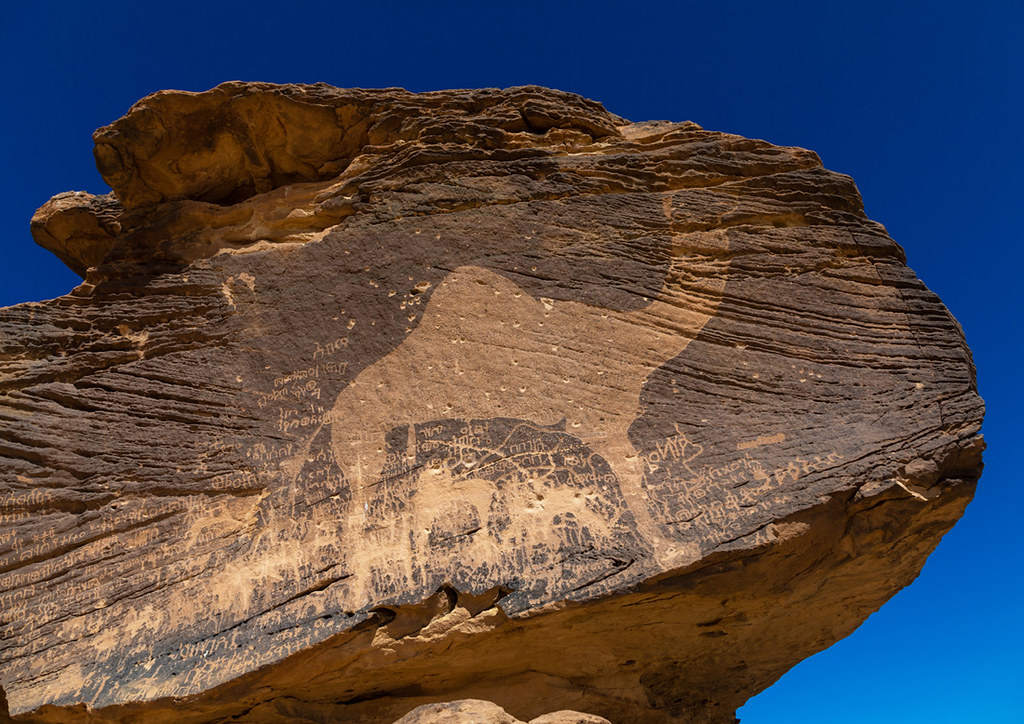A large, intricately carved rock stands prominently in the sun-baked desert landscape, set against a backdrop of clear blue sky. The rock, adorned with shades of brown and tan, features detailed etchings, including a prominent and sizable carving of a camel. The sun's rays illuminate the ancient engravings, highlighting the craftsmanship of the inscriptions that cover its surface. Though the precise location of this intriguing artifact remains unknown, its presence tells a story etched in stone, inviting contemplation of its historical and cultural significance.